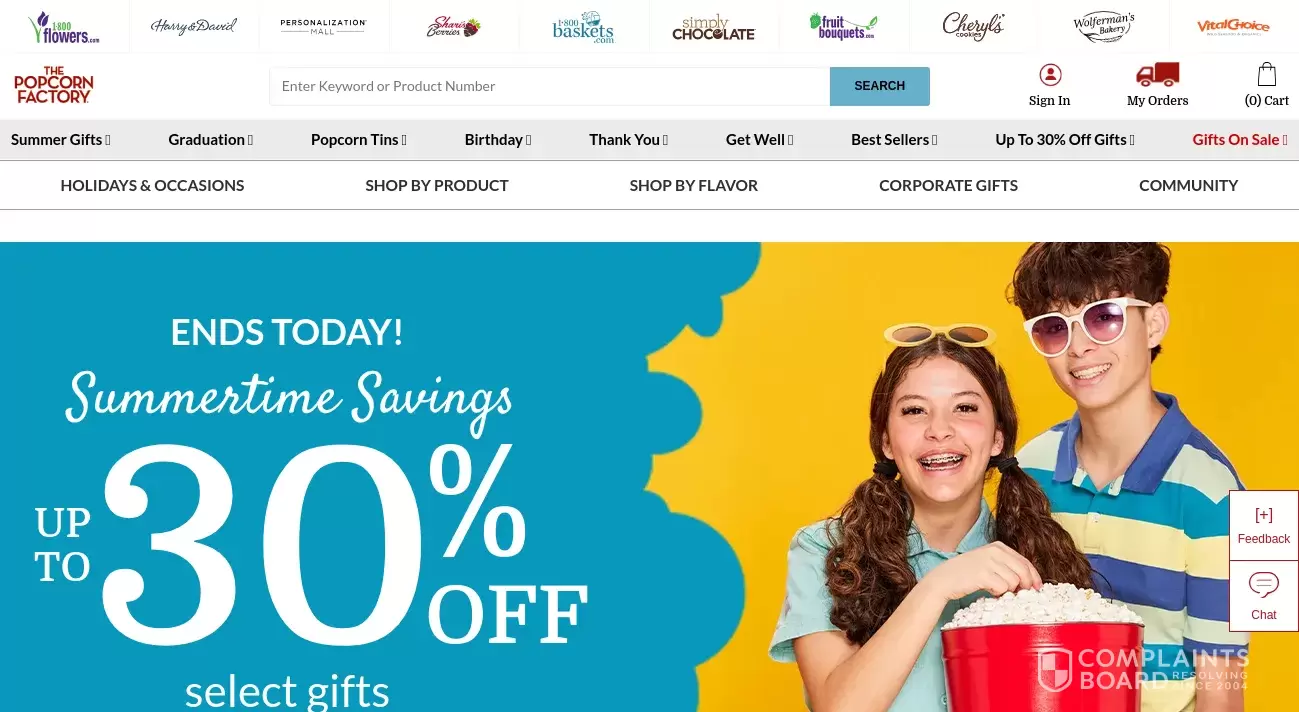This image showcases a webpage from 1800flowers.com, complete with a variety of navigation and content options. Featured prominently at the top are links to sister sites such as 1800baskets.com, Simply Chocolate, FruitBouquets.com, Cheryl's Cookies, and Wolferman's Bakery, as well as premium seafood provider Vital Choice. The header also includes options for signing in, viewing orders, checking the cart, and using the search field which prompts users to "Enter keyword or product number."

The main content area highlights several categories and promotional offers. There are sections dedicated to Easter, birthdays, thank you gifts, get well soon arrangements, and best sellers. The Easter section includes a banner offering a 31% discount on select Easter gifts, valid through Monday using the promo code 'EASTER31'. Additional navigation options allow users to shop by product, flavor, or for corporate gifts. The overall theme focuses on seasonal promotions and providing customers with a range of gifting options for various holidays and occasions.